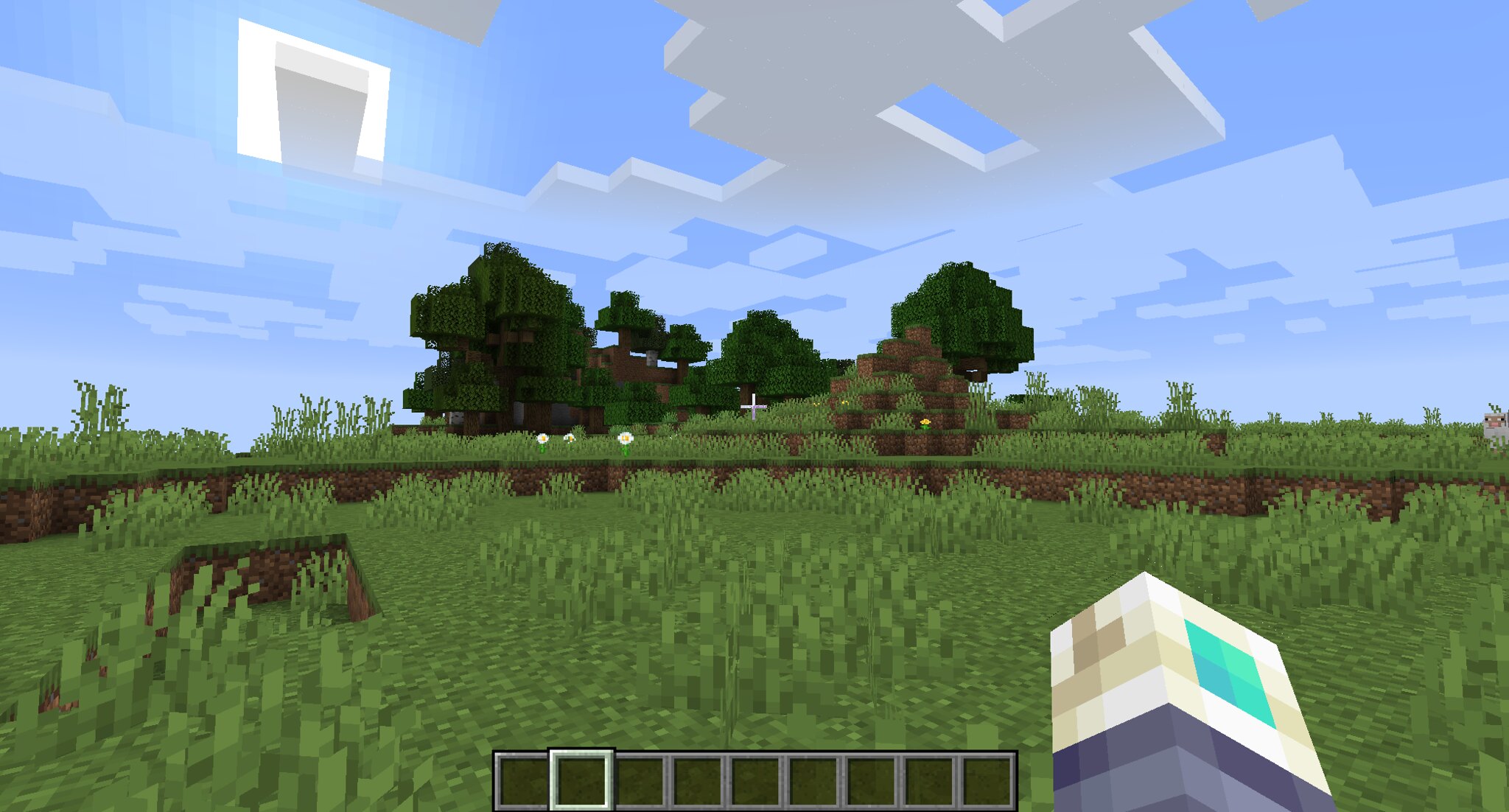This image is a digitally generated still from the video game Minecraft, showcasing a quintessential in-game scene with its signature blocky aesthetic. The scene captures a lush, grassy field extending into the distance, dotted with blocky, green-leaved trees against a backdrop of a clear blue sky interspersed with square, block-like clouds. The bottom of the screen features an inventory bar made up of nine gray squares, all currently empty except for the second one from the left, which is highlighted with a white outline. This highlights the selected but unused inventory slot. On the far right of the inventory bar, a visible avatar arm, clad in a blue shirt, extends with a pixelated white hand, indicating the player’s perspective as they navigate the landscape. Additionally, just to the right of center, a baby white sheep stands out in the grassy terrain, emphasizing the characteristic elements of Minecraft's environment. The overall visual maintains the game's iconic, blocky style, with all details including the square sun, the horizon of trees, and the cloud formations adhering to this aesthetic.